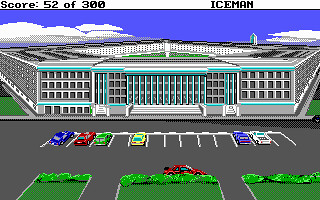This image is a screenshot from a vintage video game, likely from the 1980s or 1990s, characterized by simplistic, pixelated graphics. The scene depicts a parking lot in front of the Pentagon, recognizable by its distinctive five-sided architecture, rendered in white with light blue outlining. Above the building, the sky is dotted with three patches of clouds. 

At the top of the screen, the game's interface displays a score of 52 out of 300 in black text, with the player's name, "ICEMAN," in black, all capital letters, situated on the right side. The parking lot shows a detailed arrangement of vehicles and spaces: a blue car, a red car, a green car, an empty space, a yellow car, followed by five consecutive empty spaces, then a purple car, and a white pickup truck, with another empty space at the end—all parked facing the Pentagon. Additionally, a red car is parked sideways along a grassy section that runs through the middle of the lot. The building itself features numerous windows and several distinct angles, further enhancing the game's detailed visual representation of the Pentagon.